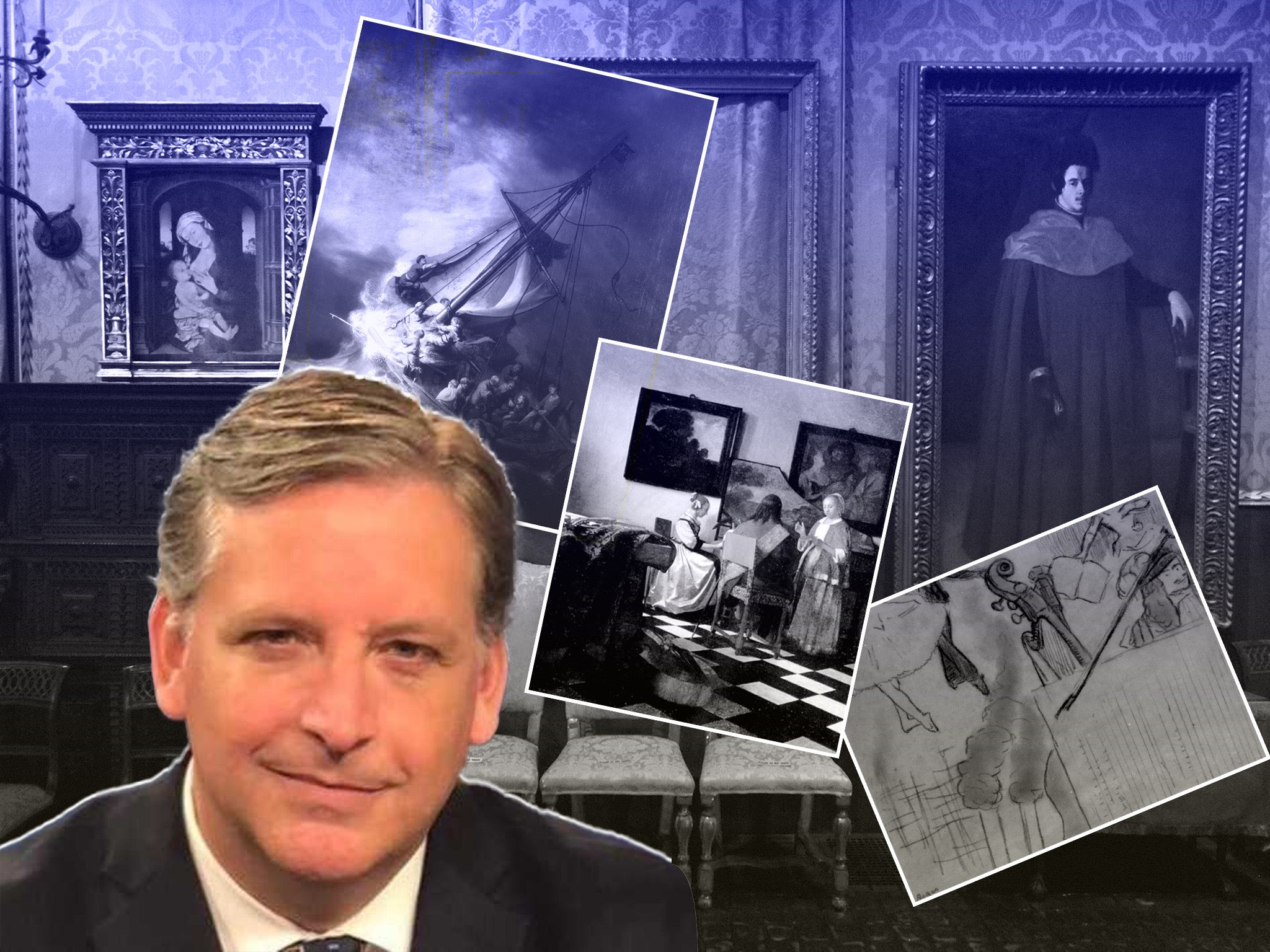The image is a collage composed of various photographs and artworks, set against the backdrop of an antique room. Dominating the scene is a large painting on the right, depicting a man, and an additional painting in the center, with another on the far left that appears to illustrate a woman nursing. In the bottom left corner of the composition, there is a close-up of a man’s face, distinctively outlined in white, suggesting he has been cut out from a different scene. The man, with short light brown hair combed back and a slight smirk, is dressed in a black suit with a white undershirt and an indistinguishable tie. Behind him, the backdrop is bluish, displaying ornate wallpaper and antique ornate frames.

Superimposed in the antique setting behind the man are three other images. The first, immediately behind him, is a blue and black depiction of a shipwreck. The middle artwork shows a scene in a room with checkerboard floors; two people are sitting while one is standing, possibly illustrating a teaching scenario, such as sewing. The farthest to the right displays what seems to be a pair of legs under blankets with nearby musical instruments, adding an enigmatic quality to the collage. Each inserted image contributes to a spectral, fragmented narrative within the antique room, drawing connections across time and scenes.